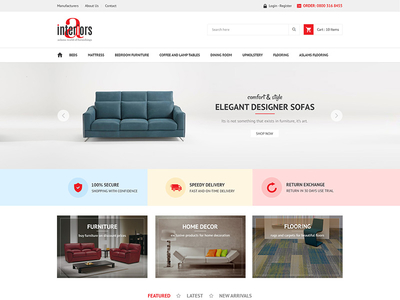This image appears to be a small screenshot of a website, predominantly featuring a white background with black text. Unfortunately, much of the text is difficult to read due to the small size, but the layout and design elements are distinguishable.

At the very top, there is a light gray menu bar that includes a phone number, as well as links for logging in and registering. Just below this, there is another menu bar that sits beside the website's logo and a search box. Adjacent to the search box, there's a shopping cart icon, indicative of an e-commerce site.

The header image prominently features a green three-seat sofa with the text "Comfort and Style: Elegant Designer Sofas," and includes additional text and a "Shop Now" button, although the smaller text is unreadable. Below this header image are three columns with bold background colors: blue, yellow, and red.

Each of these columns contains black text and small infographics in the website's red accent color. These sections provide key information such as "100% Secure," "Speedy Delivery," and "Return & Exchange." Further descriptive text accompanies these statements, but it remains largely illegible.

Additionally, there are images with links directing to various categories such as furniture, home decor, and flooring. However, similar to other parts of the image, much of the accompanying text is too small to be readable.